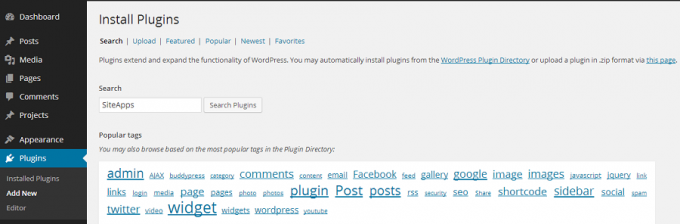This is a cropped screenshot of an application dashboard, showcasing a distinctive layout and various functionalities. The leftmost section features a black vertical navigation panel containing multiple menu items. At the very top, it displays the label "Dashboard," followed by sequentially listed items: "Posts," "Media," "Pages," "Comments," "Projects," "Appearance," and "Plugins," with the "Plugins" section highlighted by a blue bar, indicating the currently active selection.

To the right of this black column lies a prominently gray background forming an elongated rectangular area. At the top of this section, the bold heading "Install Plugins" immediately captures attention. Directly beneath this header, various tabs are listed: "Search," "Upload," "Featured," "Popular," "Newest," and "Favorites." The "Search" tab is selected, indicated by its black text, while the other options remain in blue.

Further down, explanatory text informs users that "Plugins extend and expand the functionality of WordPress." It mentions that plugins can be directly installed from the hyperlinked "WordPress plugin directory" or uploaded in zip format through another hyperlinked page.

To the left in this lower section, the word "Search" precedes a search box containing the text "white apps." Adjacent to the search box, a gray button labeled "Search Plugins" is present. Below this, a section titled "Popular Tags" displays a large white box filled with various blue, underlined tags for easy navigation.